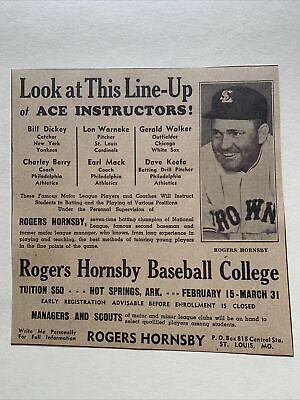The image features a vintage newspaper advertisement on a light brown paper, prominently displaying a photograph of the famous baseball player Rogers Hornsby in the upper right-hand corner. Hornsby is captured wearing a St. Louis cap and a white jersey with partially visible letters "R-O-W-N." He is smiling and looking to the left. The headline reads, "Look at this lineup of ace instructors." Below this, the text lists notable Major League players and coaches including Bill Ditkey, catcher for the New York Yankees; Charlie Berry, coach for the Philadelphia Athletics; Lon Wernke, pitcher for the St. Louis Cardinals; Earl Mack, coach for the Philadelphia Athletics; Gerald Walker, outfielder for the Chicago White Sox; and Dave Kef, batting drill pitcher for the Philadelphia Athletics. These instructors will teach students various baseball skills under Hornsby’s supervision. The advertisement is for the Rogers Hornsby Baseball College, with tuition set at $50. The college is located in Hot Springs, Arkansas, and operates from February 15th through March 31st. It advises early enrollment, with further details directed to Rogers Hornsby, P.O. Box 815, Central State, St. Louis, Missouri.